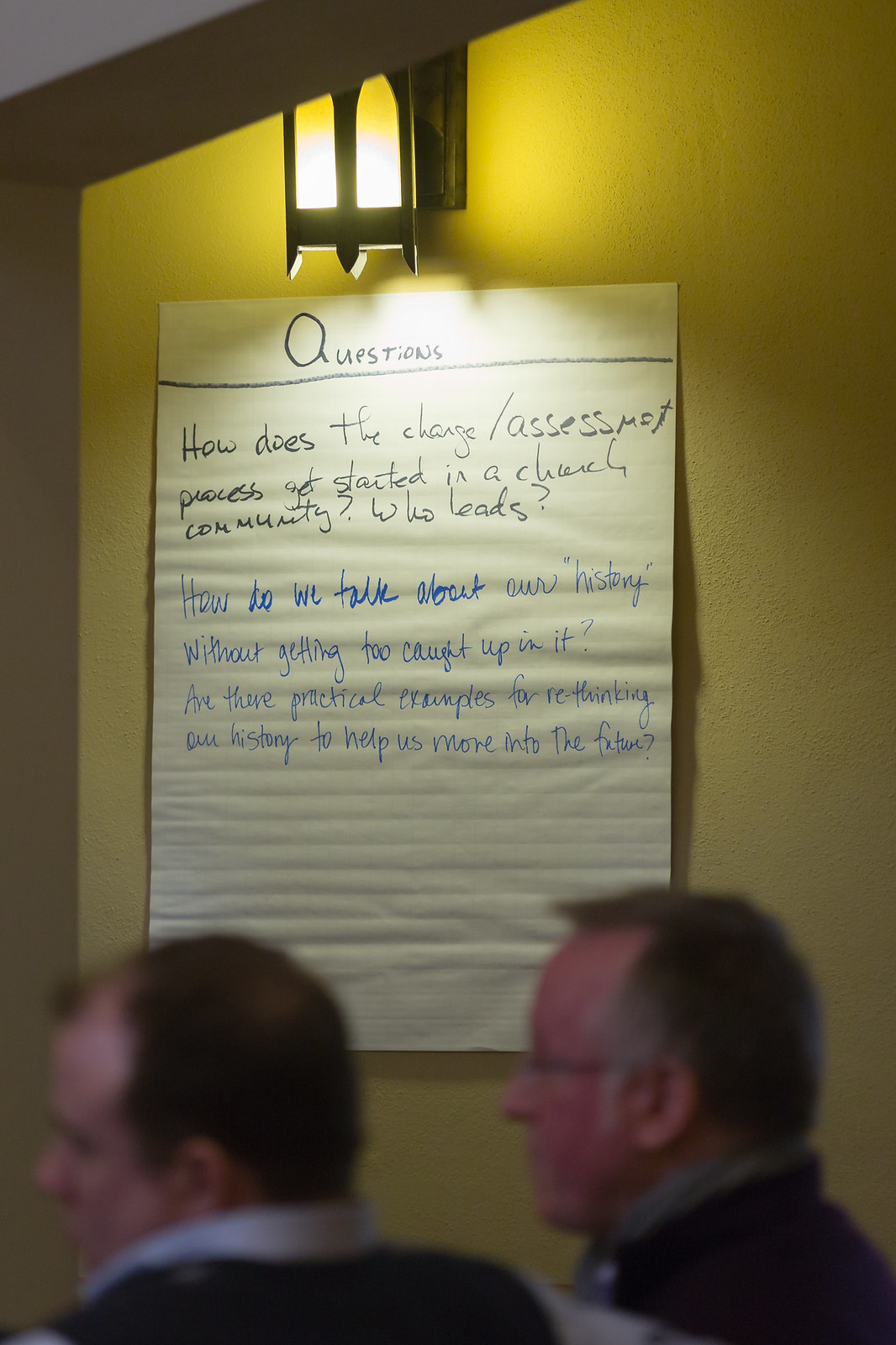This image captures a slightly blurry photograph of two men standing in profile, both looking away from the camera. They have short hair and are dressed in collared shirts paired with dark jackets or vests. The man on the right, with a hint of gray in his hair, is wearing glasses. The background features a yellow wall, with a light fixture above that shines down on a white piece of paper posted on the wall. The paper, held up by either brown or bronze fixtures, prominently displays handwritten text. At the top in black ink, it states "Questions," followed by a horizontal line across the paper. Below this, more black text asks, "How does the change/assessment process get started in a church community? Who leads?" Further down in blue text, it reads, "How do we talk about our history without getting too caught up in it? Are there practical examples for rethinking our history to help us move into the future?" Shadows cast on the yellow wall enhance the depth and atmosphere of the scene.